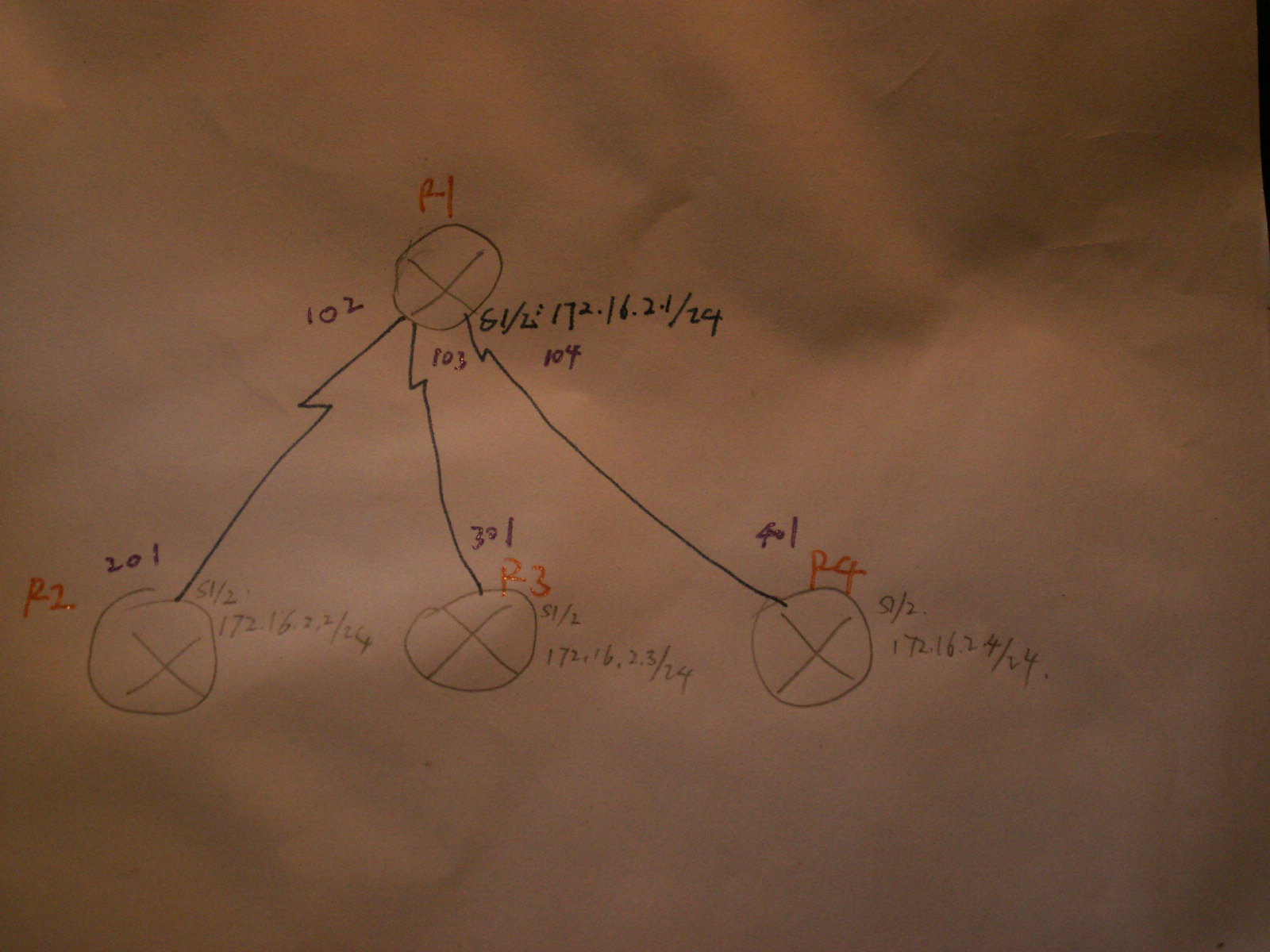The image depicts a hand-drawn graph on a brown piece of paper resembling a grocery bag. At the top, there is a circle with an X through it, marked with the number "4" in red ink above it. From this top circle, three lines resembling lightning bolts extend downwards.

The first line extends to a circle located at the bottom left, which also has an X in it. Above this bottom-left circle, the numbers "201" and "R2" are written. To the right of this circle, there are several numerical notations: "57/2," "172," "16," and "2.2/24."

A second lightning bolt-like line from the top circle descends to another circle with an X which is labeled "301" and "R3" in red ink. Next to this circle, the following numerical annotations are present: "57/2," "172," an unclear number denoted as "something," "6," and "2.3/24."

The third line also resembles a lightning bolt and travels to a circle on the bottom right with an X in it, marked "401" with "R4" written nearby. Next to this circle, it states "0/2" along with additional unidentified numbers written in ink.

Each of these elements and connections appears to signify relationships between objects, depicted with varying numerical annotations and consistent stylings of lightning bolt-like lines connecting the circles.